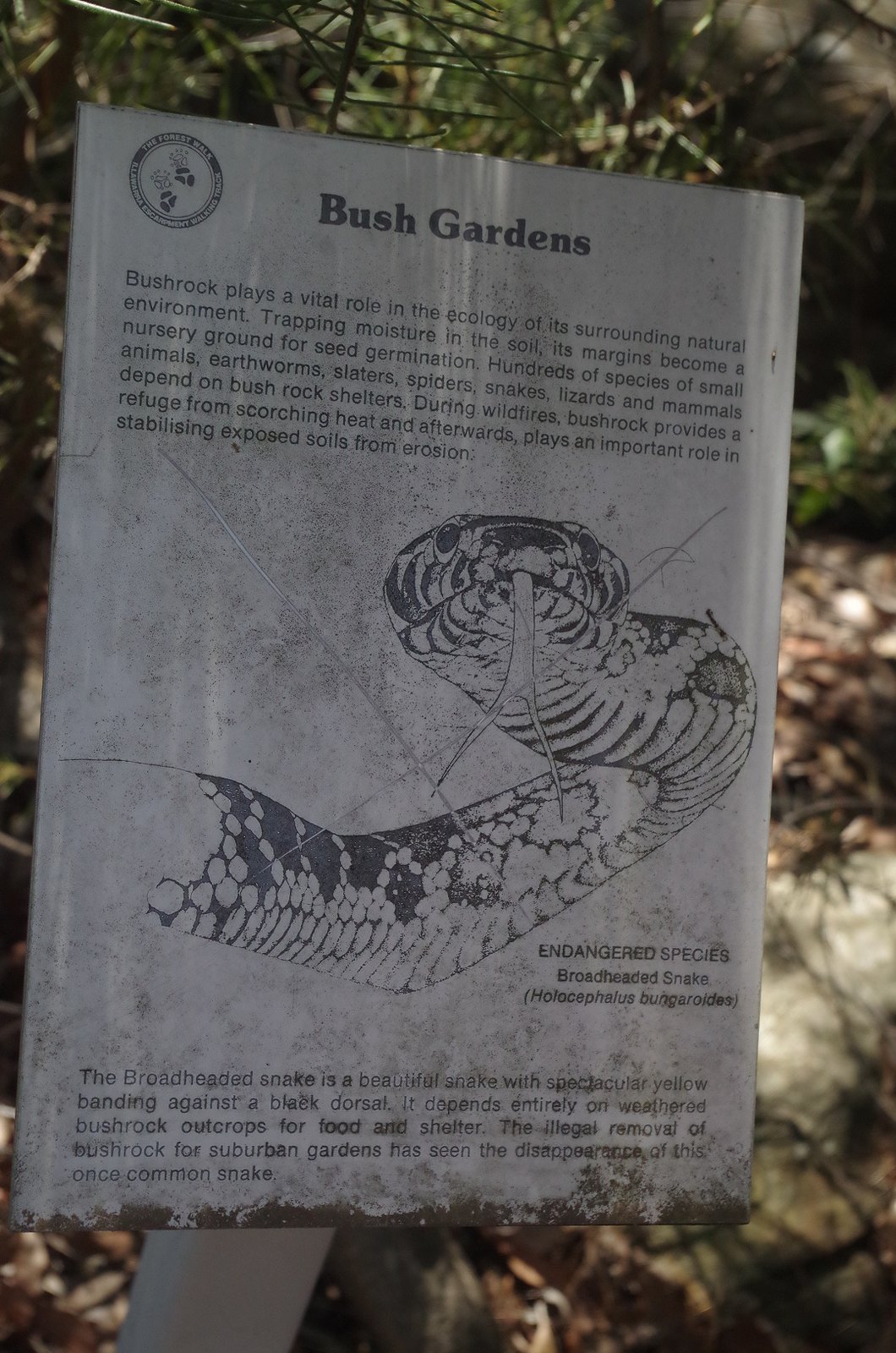The image depicts a slightly dirty and rusted grey metal plaque mounted on a white pillar, likely situated in a garden or zoo, with a backdrop of green foliage, brown earth, and leaves. The top of the plaque prominently reads “Bush Gardens” in bold text. Central to the plaque is an etched image of a black and white broad-headed snake, with its body extending from the left to the center right and its head positioned in the center right, tongue protruding.

The primary text explains the importance of bush rock in the ecosystem: “Bush Rock plays a vital role in the ecology of the surrounding natural environment, trapping moisture in the soil. Its margins become a nursery ground for seed germination. Hundreds of species of small animals, earthworms, spiders, snakes, lizards, and mammals depend on bush rock shelters. During wildfires, bush rock provides a refuge from scorching heat and afterwards plays an important role in stabilizing exposed soil from erosion.”

Further details about the snake, identified as an endangered species, are included at the bottom of the plaque: "The broad-headed snake (Holocephalus bungaroides) is a beautiful snake with spectacular yellow banding against a black dorsal. It depends entirely on weathered bush rock outcrops for food and shelter. The illegal removal of bush rock for suburban gardens has seen the disappearance of this once common snake."